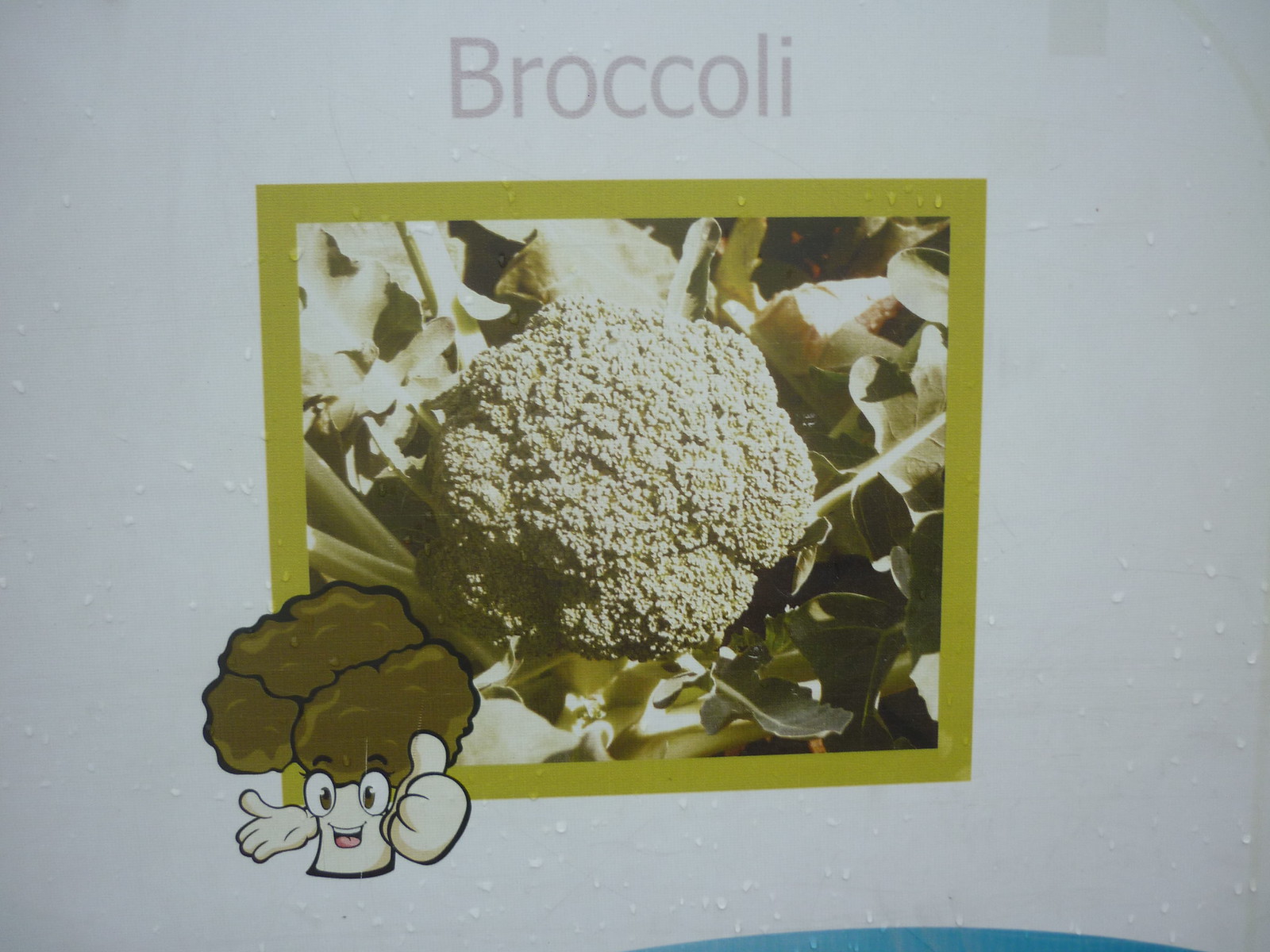The image is a color photograph with a white background, featuring the word "Broccoli" in light mauve text across the top. In the center, there is a slightly washed-out rectangular photograph of a piece of broccoli, bordered by a consistent lime green frame. The broccoli appears muted in color, suggesting either an applied filter or a peculiar lighting condition. Surrounding the broccoli are undulating leaves, adding a dynamic touch to the scene.

In the bottom left corner of this green-framed photograph, there’s an anthropomorphized cartoon broccoli character. This little character has a stem with a smiling face that includes two oval eyes, playful eyebrows, and a pink tongue. One of his hands is outstretched with the palm facing up, while the other hand is clenched into a fist giving a thumbs-up, possibly wearing gloves. This cartoon broccoli adds a cheerful element to the image.

The background includes random water droplets, suggesting a likely refrigerated environment, and there's a bluish hump in the bottom right corner. Furthermore, a small piece of sellotape is visible at the top right, hinting the image might be affixed to a surface like a fridge or a door.